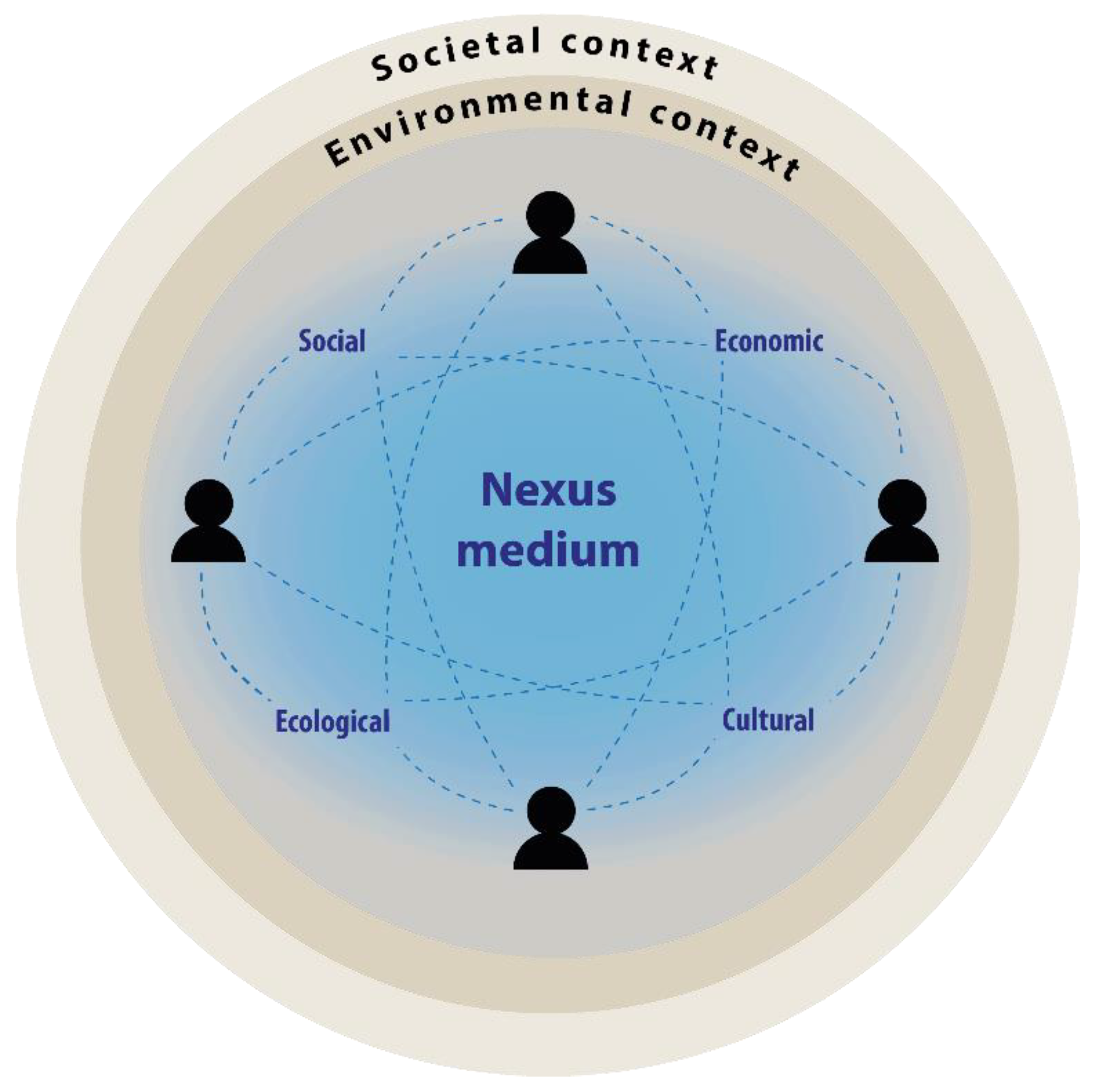The image is a highly detailed circular digital poster featuring three nested concentric circles. The outermost circle is light grey and labeled "Societal Context" in black text at the top. Within this is a light brown circle with the wording "Environmental Context" also in black at its top edge. The innermost circle is primarily light blue, deepening in color towards the center, and contains four black human silhouette figures positioned at the cardinal points: top, bottom, left, and right. These figures are interconnected by blue dotted lines, forming a pattern reminiscent of a molecule or a floral arrangement. Between these figures, key terms such as "Social," "Economic," "Cultural," and "Ecological" are inscribed in black. At the very center of this intricate design, the phrase "Nexus Medium" is prominently displayed in large blue text, highlighting the interconnectedness represented in the diagram.